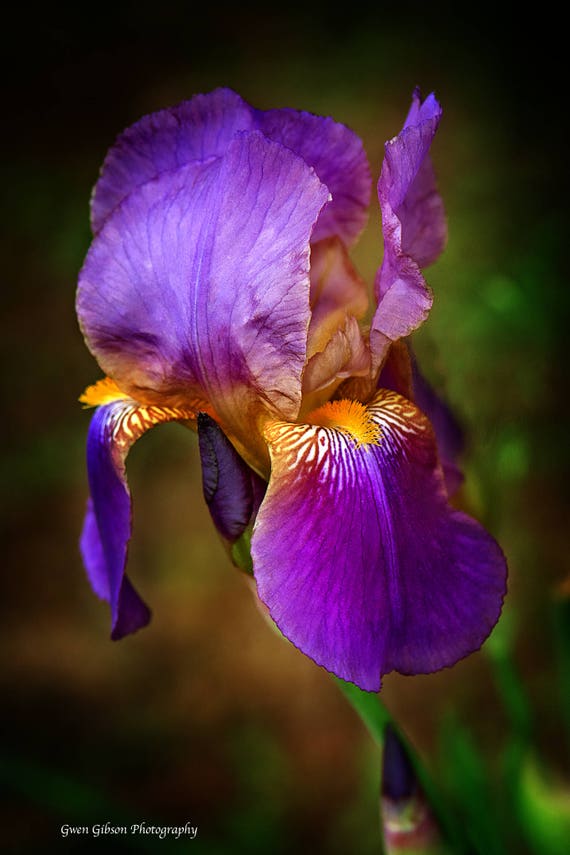This portrait-layout photograph by Gwen Gibson captures an exquisite close-up of an orchid. Central to the image are the flower's delicate petals, showing striking shades of purples, indigos, and blues. The petals have intricate veins, with some featuring yellow fur-like structures emerging from their base. The flower has six petals: four extend vertically while two fold over, revealing a mix of orange, white, and brown hues at the core. Surrounding the flower is a blurry, mottled background that shifts from light green at the center to darker green and black towards the edges, suggesting out-of-focus leaves or vegetation. A green stem can be faintly discerned, supporting not just the main flower but also hinting at another blossom nearby. The lower left corner of the image includes a white-font credit to Gwen Gibson photography, ensuring the artist's recognition for this beautifully detailed and vividly colored botanical portrait.